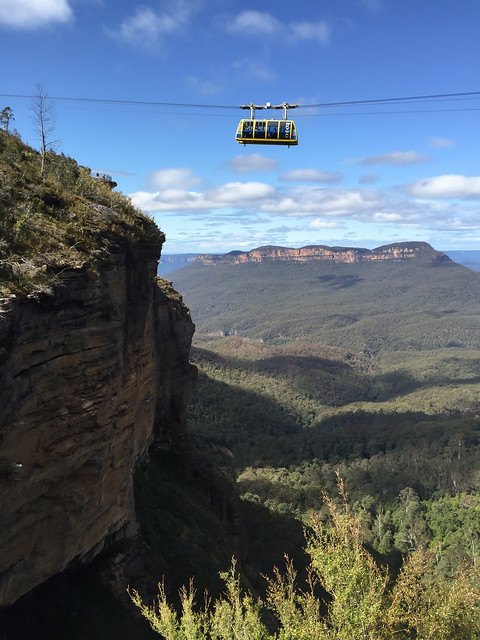This captivating image captures a dramatic and beautiful mountain landscape under a bright blue sky adorned with fluffy white clouds. In the center of the image, a yellow gondola with large windows glides across a canyon, suspended from sturdy cables. The gondola seems to be carrying passengers, offering them spectacular views of the rugged terrain below. The scene is bathed in daylight, and the sunlight casts a shadow of the gondola onto the ground far below. The left side of the image is dominated by a formidable cliff which appears to drop sharply, possibly hundreds of feet, into a verdant valley filled with greenery, rolling hills, and trees. One noticeable tree near the cliff edge is bare of leaves, adding to the dramatic effect. This blend of natural beauty and high-altitude adventure creates a striking and somewhat daunting visual, especially for those uneasy with heights.